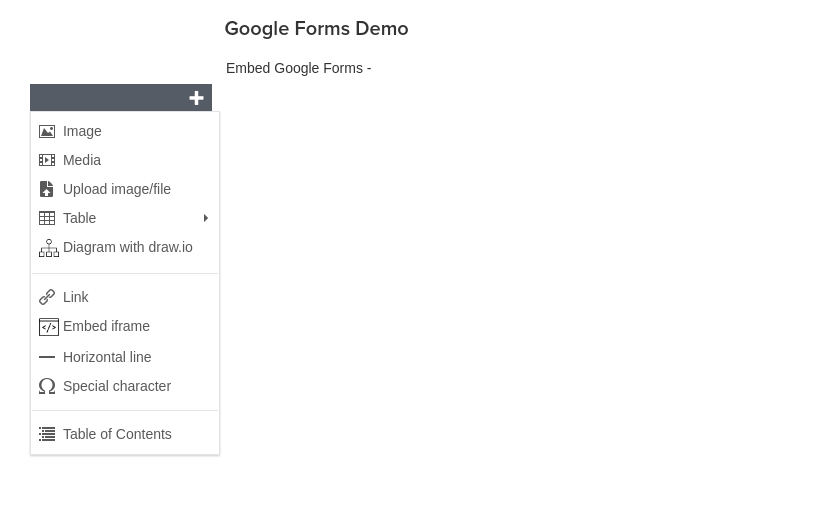A screenshot of a computer screen displaying a tutorial slide titled "Google Forms Demo" at the top. The slide appears to be part of a PowerPoint presentation, guiding users on how to embed Google Forms. Below the main header, smaller text reads "Embed Google Forms." The screen features a pop-up menu with a black bar at the top showcasing a plus icon. 

The menu lists various interactive elements for inclusion, such as:
- **Image**
- **Media**
- **Upload Image or File**
- **Table** (with an option to design the table by dragging through to specify the number of cells)
- **Diagram with draw.io** (accompanied by an icon illustrating an organizational chart)
- **Horizontal Line**
- **Link**
- **Embed iframe**
- **Special Character** (indicated by an omega symbol)
- **Table of Contents**

The overall layout suggests a step-by-step guide on enhancing a Google Form through various embedded elements, likely aimed at users looking to create more sophisticated and interactive forms.